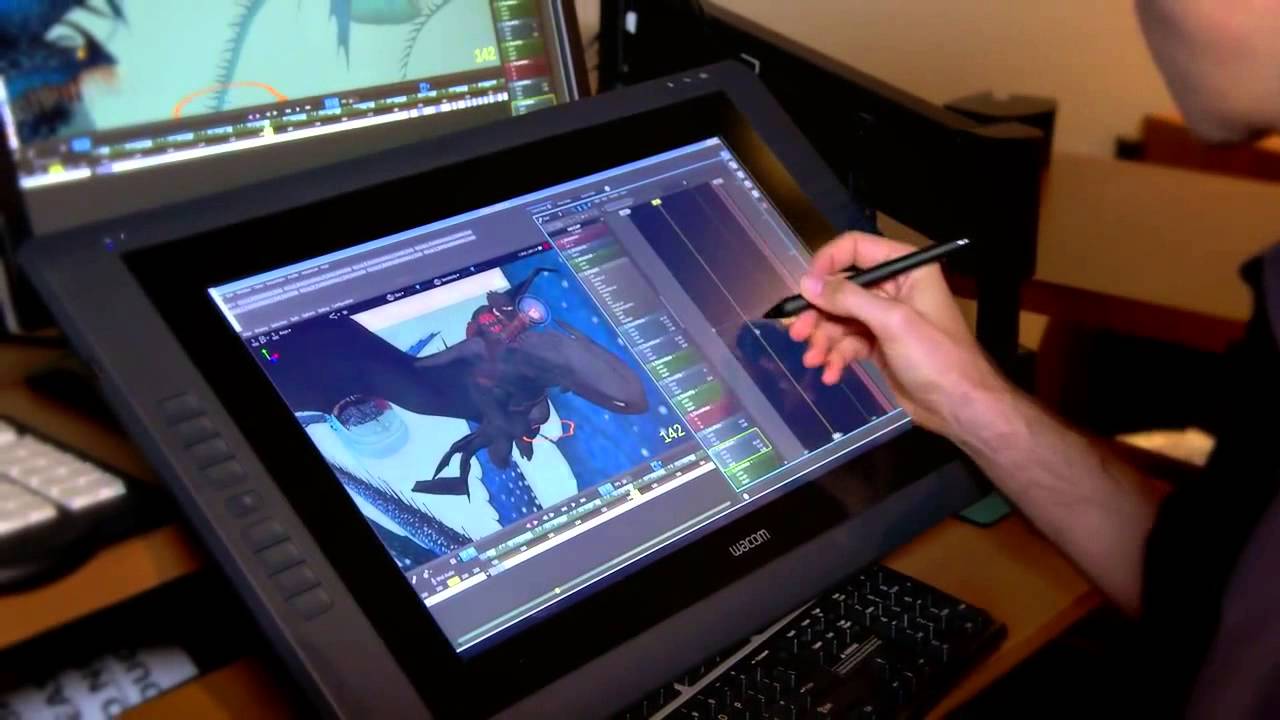The image shows an angled view of an animator at work, focusing on his right hand as he uses a black stylus to draw on a large Wacom drawing tablet. His hairy forearm is visible, extending just past the elbow, supporting the inference that he is a male. The drawing on the screen depicts a person riding the back of a black dragon, with some circular element that could indicate a superpower or special effect tied to the scene. Above the drawing tablet is another larger monitor displaying the same image for easier visibility. Both screens, along with a black keyboard and another partial view of a keyboard with white keys and a black plastic outline, are all situated on a brown desk. The animator's chin is slightly visible in the shot, but his face remains out of the frame.